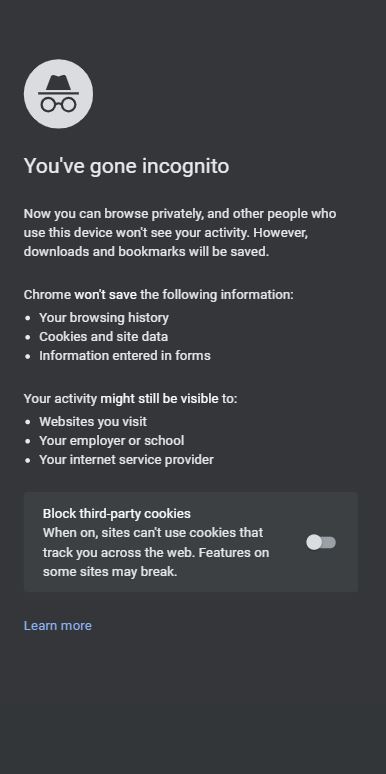The web page displays the message that appears when a user selects to browse in Google Chrome's incognito mode. The background is a blend of purple and grey hues. At the top of the page, the Google Chrome incognito icon is prominently featured, consisting of a line drawing of a fedora and spectacles, rendered in black on a white background.

Just below the icon, a heading reads "You've gone incognito." The accompanying message explains that users can now browse privately and other people using the device won't see their activity, although downloads and bookmarks will still be saved. 

Further information is presented in a structured format with line spacing and bullet points. The message clarifies that Chrome won't save the following information:

- Your browsing history
- Cookies and site data
- Information entered in forms

An additional note specifies that your activity might still be visible to:

- Websites you visit
- Your employer or school
- Your internet service provider

Below this, there is a toggle box for "Blocked third-party cookies." When this setting is on, it prevents sites from using cookies that track the user across the web, although this might cause some sites to malfunction. The on-off indicator is positioned on the left side.

At the bottom of the page, there is a "Learn more" link in pale blue font, providing further information about incognito mode.